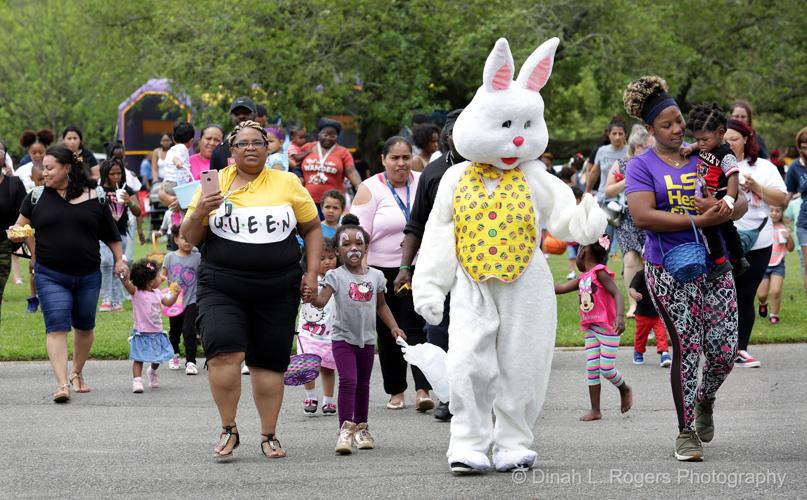In the foreground of this vibrant image set in a park, a group of people, composed primarily of African American women and children, gather on an asphalt path. Dominating the center, an individual dressed as an Easter Bunny captivates attention with a white and pink bunny costume, complete with a large head and a yellow vest adorned with small, colorful designs and Easter eggs. To the left, a heavy-set black woman with glasses holds a smartphone in a pink cover with her right hand, wearing black and yellow clothes that spell out "Queen," while holding the hand of a young child with her left. Surrounding them are about 35 people of various ages, although none appear elderly. The children, some with painted faces resembling bunnies, carry Easter baskets, hinting at an ongoing Easter egg hunt. In the background, the park’s grass and multiple trees contribute a lush green scene, and a bounce house suggests further festivities. Splashes of vibrant colors—pink, yellow, white, purple, orange, red, and light blue—add to the lively atmosphere. The crowd seems unified as they move in the same direction, capturing the essence of this Easter event. An inscription in white letters at the bottom right corner credits the picture to "Dinah L. Rogers Photography."